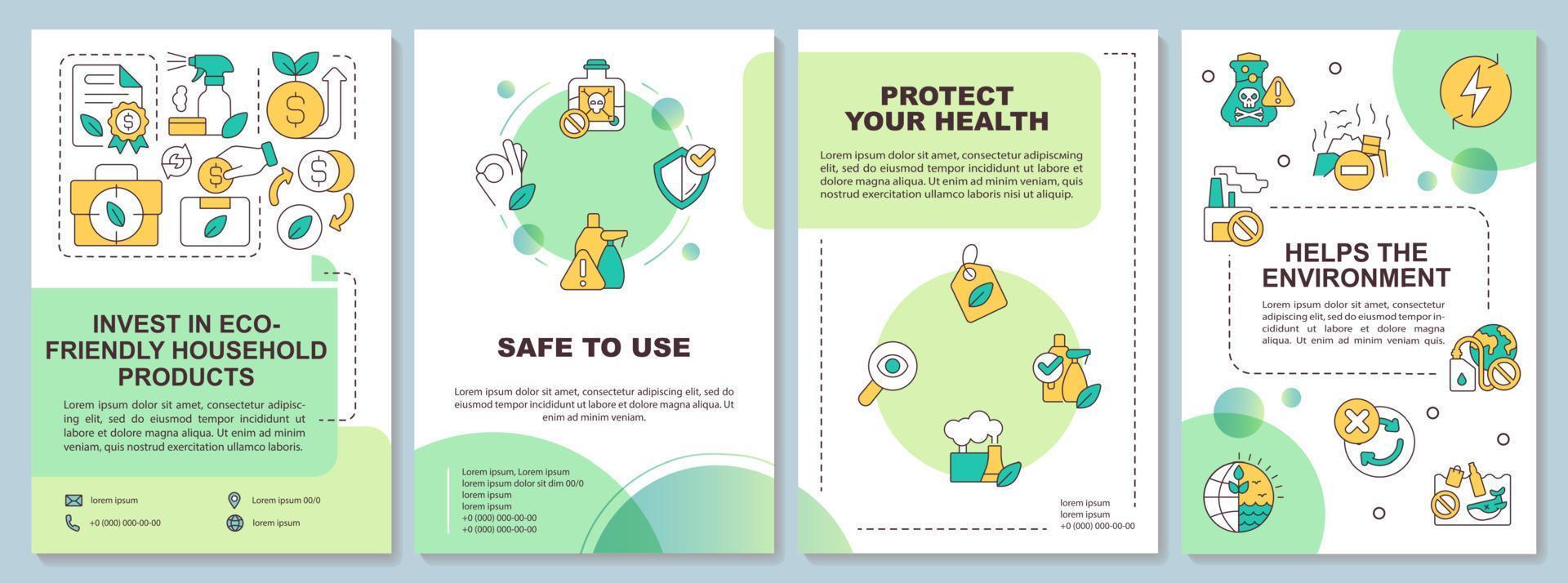The image features a rectangular series of four vibrant informational posters set against a gray background. Each poster is side by side in a single row, prominently displaying a public service announcement about eco-friendly household products. The first poster, predominantly in gold and greens, encourages investment in eco-friendly household products and includes a diagram with a dollar sign and gold graphics. The second poster emphasizes safety, with checkmarks indicating safe actions and symbols showing what to avoid, highlighting the safety benefits of these products. The third poster, on a green background, focuses on health protection, detailing how eco-friendly products can benefit your health, and includes visuals related to health and labeling. The fourth and final poster highlights environmental benefits, featuring images of a factory emitting smoke and a beaker with a skull and crossbones, indicating the harmful substances to avoid. Bright and colorful, the posters predominantly use gold, green, and light green hues, creating a visually engaging and informative presentation.